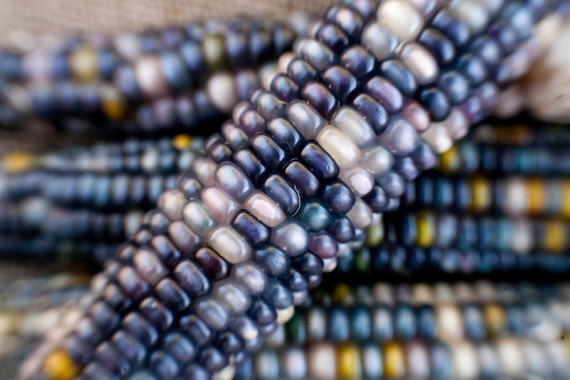The image features a close-up, diagonal shot of a uniquely colored corn cob, with its kernels displaying a striking blend of black, white, and a few yellow pieces interspersed. The cob is long and slender, prominently focused in the middle, with its shiny, almost pearlescent kernels exuding a magical, iridescent quality. The backdrop consists of three similarly exotic corn cobs, heavily blurred, enhancing the depth and emphasis on the foreground. This photographic arrangement, lying against a tan background, is crisp and detailed only in the central focus area of the main corn cob, making it suitable for a high-quality farming magazine or seed catalog. The overall visual effect suggests these cobs are freshly shucked and naturally vibrant in their coloration, rather than artificially dyed.